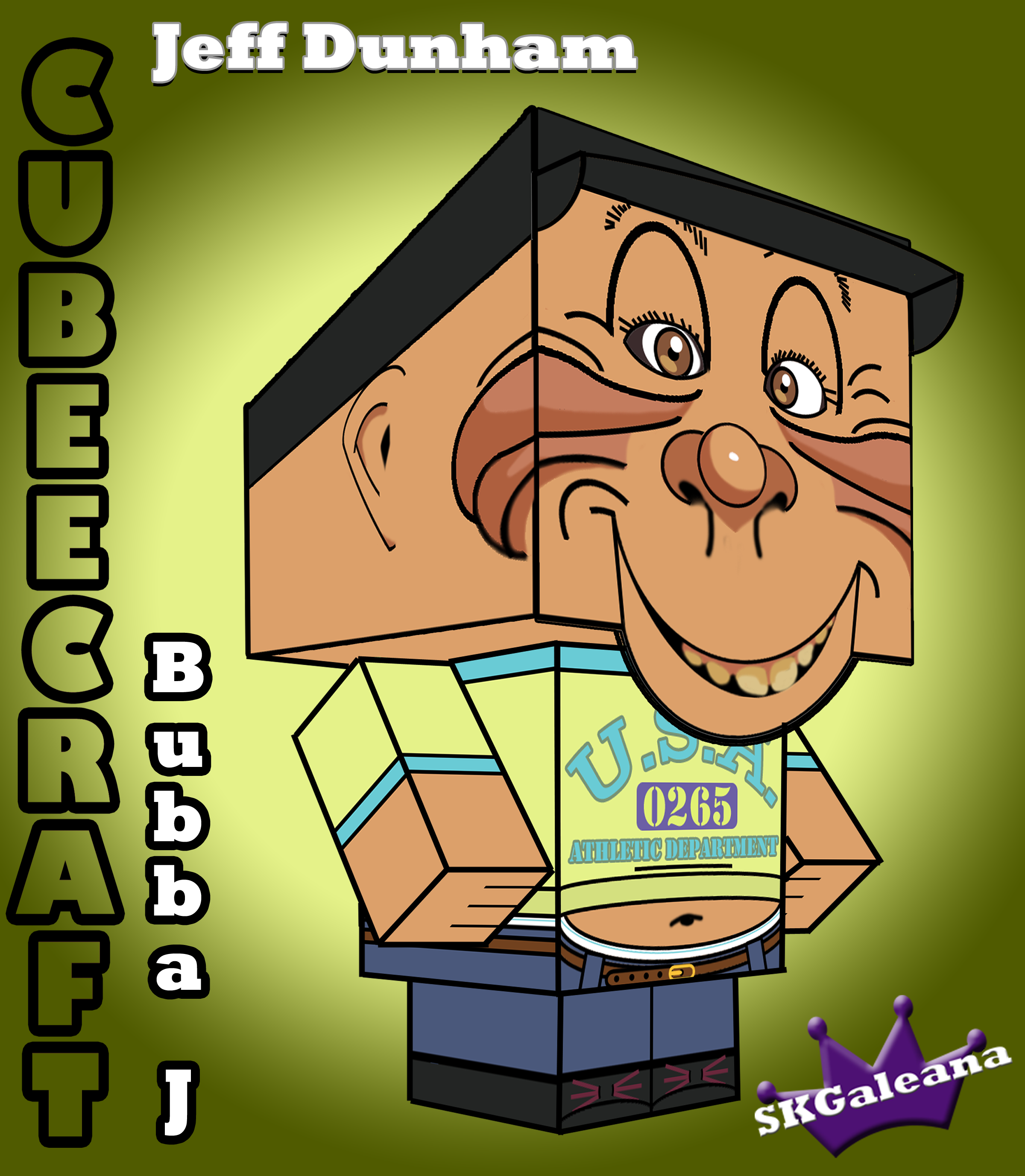The image is a detailed digital illustration of a cube-like cartoon character resembling a stick figure with a square box for a head. The character is facing at an angle to the right, sporting a black hat and a big goofy smile. Featuring angular, lined cheeks, a round nose, and brown eyes, the character's skin is brown. He wears a yellow and blue t-shirt with the text "USA 0265 Athletic Department," revealing a midriff typical of an overweight figure. His blue jeans are secured with a brown belt, and he has black shoes with red laces. The background of the image is green. In the upper left corner, white text reads "Jeff Dunham," while down the left side, black text spells "Cubeecraft" with "Bubba J" in white letters beneath it. In the lower right corner sits the text "SK Galeana" overlaid on a purple crown.